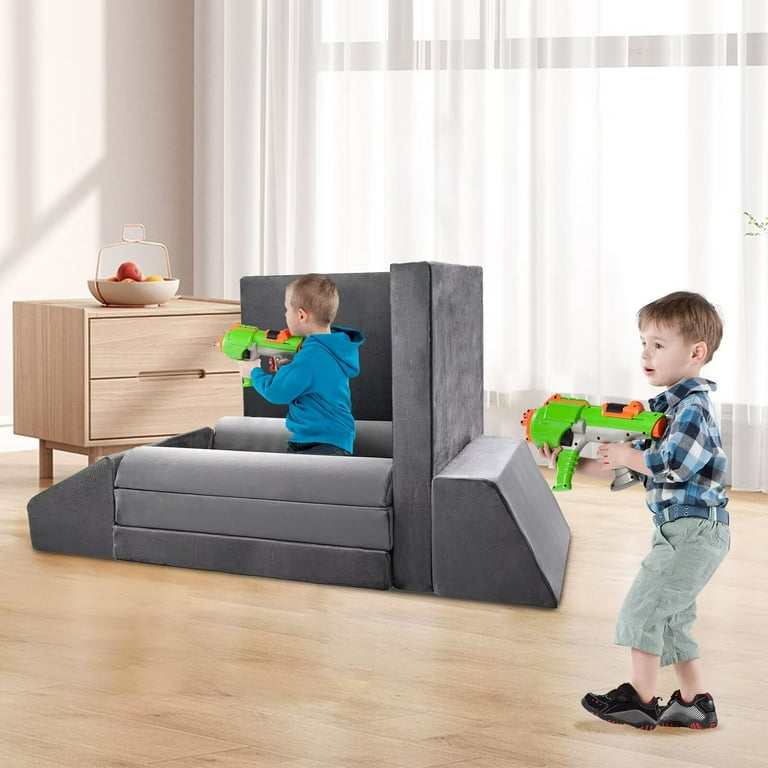In a bright, open living room bathed in natural light from a floor-to-ceiling window adorned with sheer white curtains, two young boys engage in an imaginative play battle with NERF blasters. The room features modern, minimalistic decor with taupe or light gray painted walls and a spacious light-colored hardwood floor. Sparse yet tasteful furnishings include a light wood two-drawer nightstand topped with a white bowl filled with colorful fruit, subtly adding to the playful ambiance.

One boy, possibly around four or five years old, is stationed on the left side of the photo. Clad in a teal hoodie, he sits within a fort ingeniously constructed from various wedge-shaped, bolster-shaped, and flat gray cushions, likely repurposed from an unseen sofa. He aims his green and orange NERF blaster at the nightstand, fully absorbed in his game. The second boy, perhaps slightly younger or the same age, stands on the right side of the image. Dressed in a blue, black, and white plaid long-sleeved shirt, gray three-quarter length pants, and black sneakers, he too holds a NERF blaster and gazes out of the frame, ready for whatever imaginative scenario comes next. The photograph captures the essence of childhood creativity and joy within a sophisticated, well-lit modern living space.